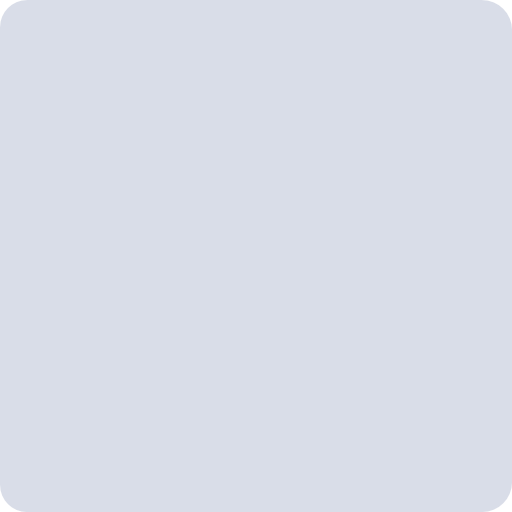A peculiar image presents itself as a vast and featureless expanse of gray. The space is marked by a subtle gradient transitioning from a darker gray at the top to a slightly lighter gray at the bottom, adding the faintest hint of depth. The shape of the image is akin to an icon on an iPhone, boasting soft, rounded corners that suggest modern design aesthetics. These rounded edges might indicate transparency, seamlessly blending into the white background, thus rendering any edge detailing invisible. Essentially, this image is a cropped screen capture of an empty gray field, meticulously devoid of any noteworthy elements.